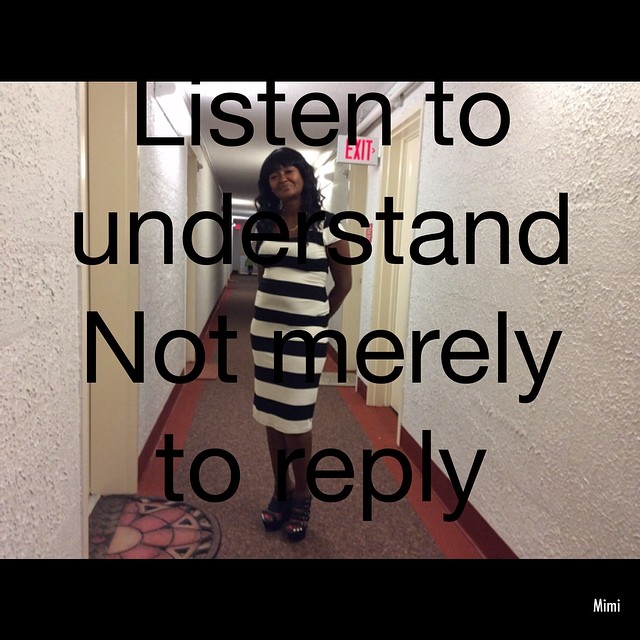This photo features an African-American woman standing confidently in the middle of a long hallway, possibly part of an apartment building or a hotel, given the mix of exit signs, doors, and welcome mats. She is wearing a black and white striped dress with horizontal stripes, short sleeves, and a scoop neckline, which falls just past her knees. Her long black hair complements her smirk, adding a touch of intrigue to her expression.

The hallway itself has light-colored, textured walls, possibly resembling a popcorn ceiling finish. The doors lining the hallway are off-white, some adorned with welcome mats, indicating a more residential setting. The floor features a border in a burnt orange-ish red hue with a speckled center, possibly in brown or burgundy tones. 

Overlaying the image are four lines of black text reading, "Listen to understand, not merely to reply," emphasizing a meaningful message. The photo is bordered in black at the top and bottom, with the name "Mimi" written in white at the bottom border.